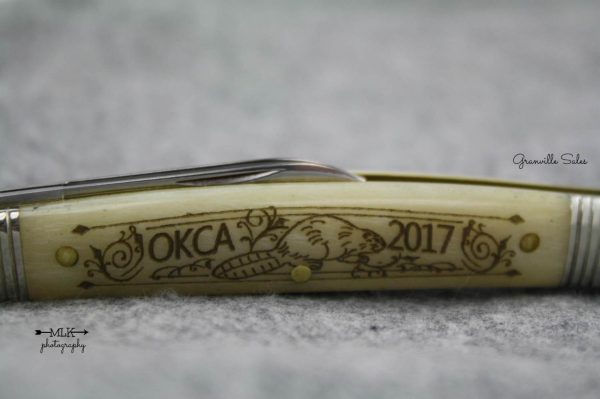This is a detailed close-up photograph of a folded single-blade pocketknife. The handle, which is an off-white or ivory color, features an engraving that reads "OKCA 2017” with an intricate line drawing of a beaver nestled between the text. Surrounding the beaver are decorative lines above and below the text, as well as some swirl lines to the left and right, and a small depiction of ground and a bush. The blade itself is silver and folded into the handle, with the notch for opening visible. The ends of the handle are silver, and the pocketknife rests on a marble gray countertop.